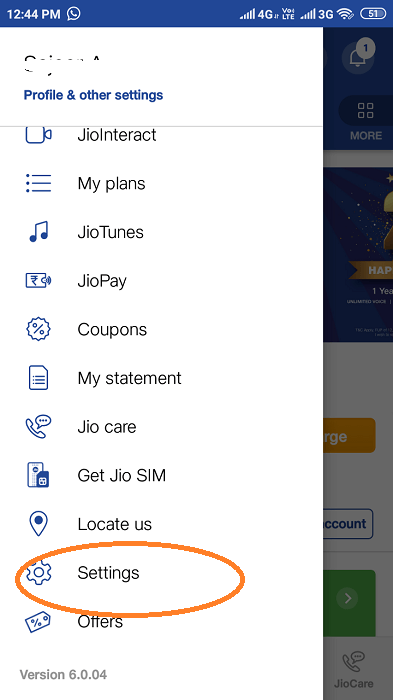Screenshot Caption:

This image is a screenshot captured at 12:44 p.m. as indicated by the white text on a blue bar at the top of the screen. The bar features various icons including a phone signal indicator, displaying both 4G and 3G symbols, a Wi-Fi symbol, and a battery indicator showing 51%.

Below this bar, a menu overlaid on the image is displayed against a white background. The menu is titled in blue text as "Profile and Other Settings," with the following options listed in black text accompanied by blue icons:
- "JioInteract" featuring a camcorder icon.
- "My Plans" with a list icon.
- "JioTunes" displaying a music note icon.
- "JioPlay" represented by a TV icon.
- "Coupons" with a circle containing a percentage sign.
- "My Statement" denoted by a paper icon.
- "JioCare" featuring a phone icon with a speech bubble.
- "Get Jio SIM" illustrated with a SIM card icon.
- "Locate Us" indicated by a location pin icon.
- "Settings" with a cogwheel icon.
- "Offers" symbolized by a price tag icon.

At the bottom of the menu, in gray text, it states "Version 6.0.04."

The background of the image is dimmed out but discernible. A white and blue notification bell icon with the number one is visible next to four white boxes labeled "More". There is a partially visible banner with blue and gold colors, only showing the word "Gold" and partly obscured festive text. Moreover, the background features a white section with a gold and white box, a blue and white box, and a green section, partially displaying a phone and speech bubble icon labeled "JioCare".